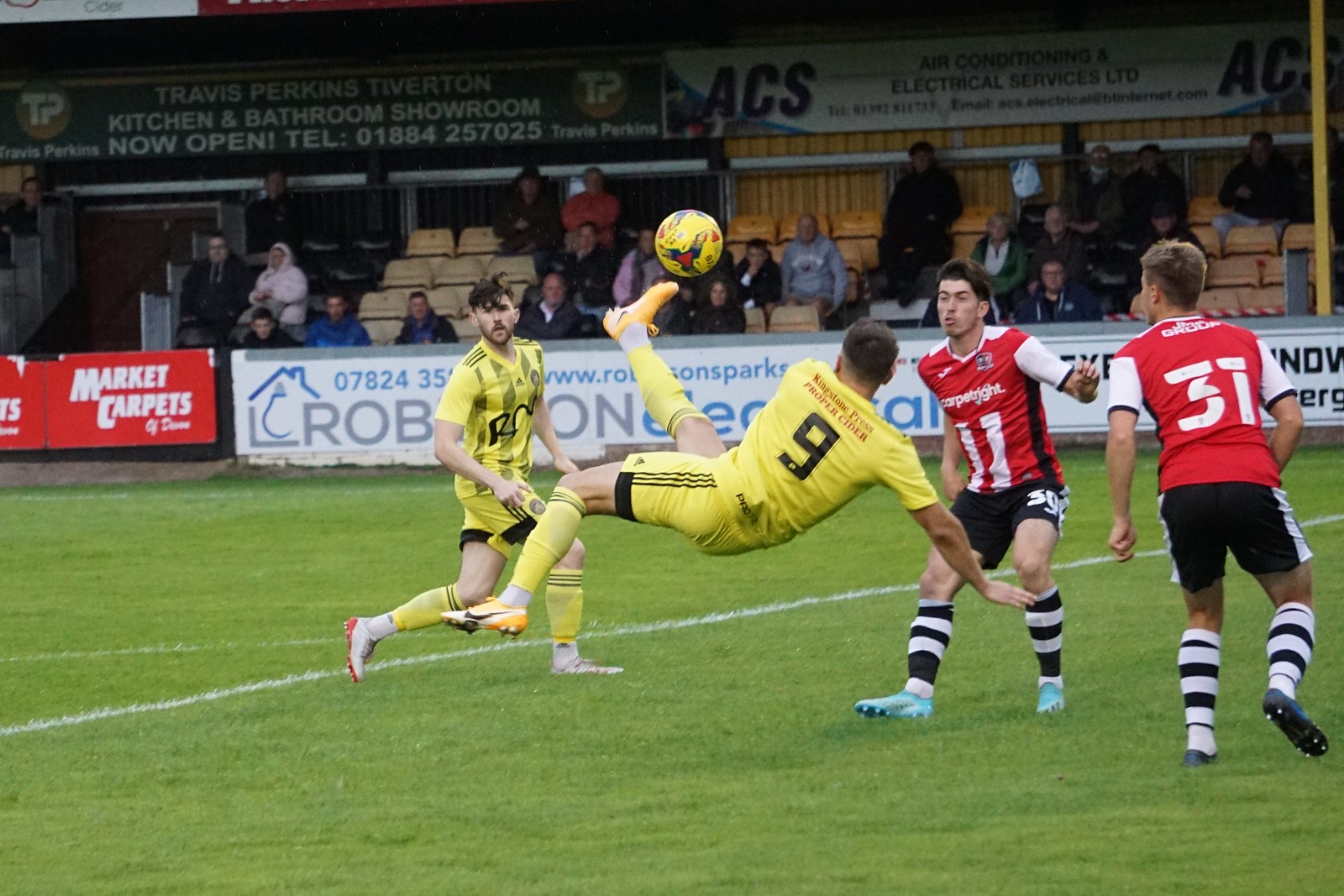The image captures a dynamic moment during a soccer match on a green field with white lines. In the foreground, a player in a yellow jersey with black trim, marked with the number 9, is mid-air performing a lateral kick. His body is twisted, one arm outstretched for balance, and one foot is actively striking a yellow soccer ball, decorated with black, red, and white markings, while the other foot dangles mid-air. His attire includes yellow shorts with black stripes and yellow socks with black accents. 

Nearby, another player in a matching yellow jersey and black-trimmed shorts, wearing shoes in red and white hues, is running towards the airborne player, appearing to lunge or brace for impact. On the right side of the frame, two opponents donning red jerseys with white sleeves and black shorts, marked with numbers 11 and 31 respectively, are engaged in the scene. Both players sport black and white socks, with one wearing blue shoes and the other black and blue ones.

In the background, spectators fill an array of black, tan, and yellow seats, framed by a white and silver cage structure. Various advertisements and banners in white, red, blue, and green, featuring texts like "market carpets", "Travis parking, Tibberton, kitchens and bathrooms, showroom, now open", and "ACS air conditioning and electrical services, LTD" are visible around the stadium. Black and yellow walls provide the backdrop for these signs, adding to the vivid atmosphere of the match. The crowd is animated, predominantly dressed in black, contributing to the excitement captured in this action-packed moment.